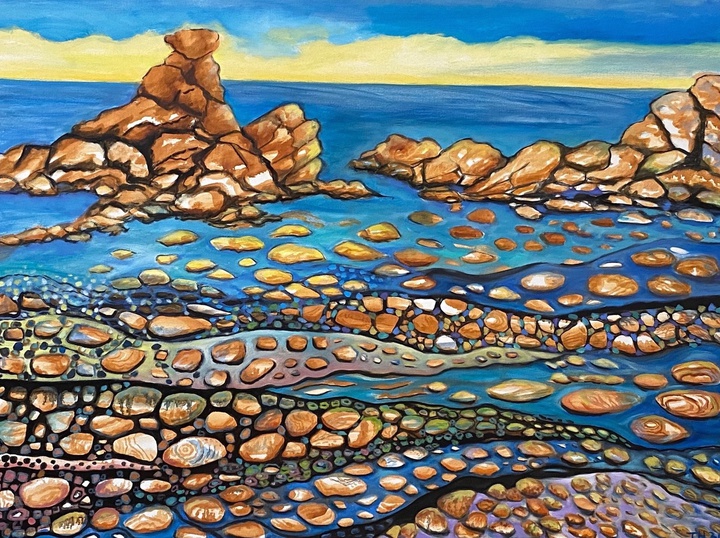This painting depicts a serene rocky beach scene with a richly detailed interplay of colors. At the top, the sky transitions from a light to darker blue, with a yellow horizon melding into scattered clouds. Below this, the vividly blue water reflects the tranquil ambiance of the scene. Dominating the left side of the image is a tall, stacked formation of brown boulders that seem to reach towards the sky, forming a triangular silhouette. Just right of this formation, another cluster of boulders stands amidst a scattered array of circular stones, which are partially submerged in the water. Notably, these boulders are characterized by deliberate separations and distinct color variations, ranging from browns with touches of white and orange to other subtle hues. The foreground is animated by segmented wave ripples and rock pathways made of multicolored bands, including blues, purples, pinks, and even dark shades. The careful arrangement of lines and color shifts in these sections adds a dynamic flow, guiding the viewer's eye from the calm sea to the intricate details along the water's edge.